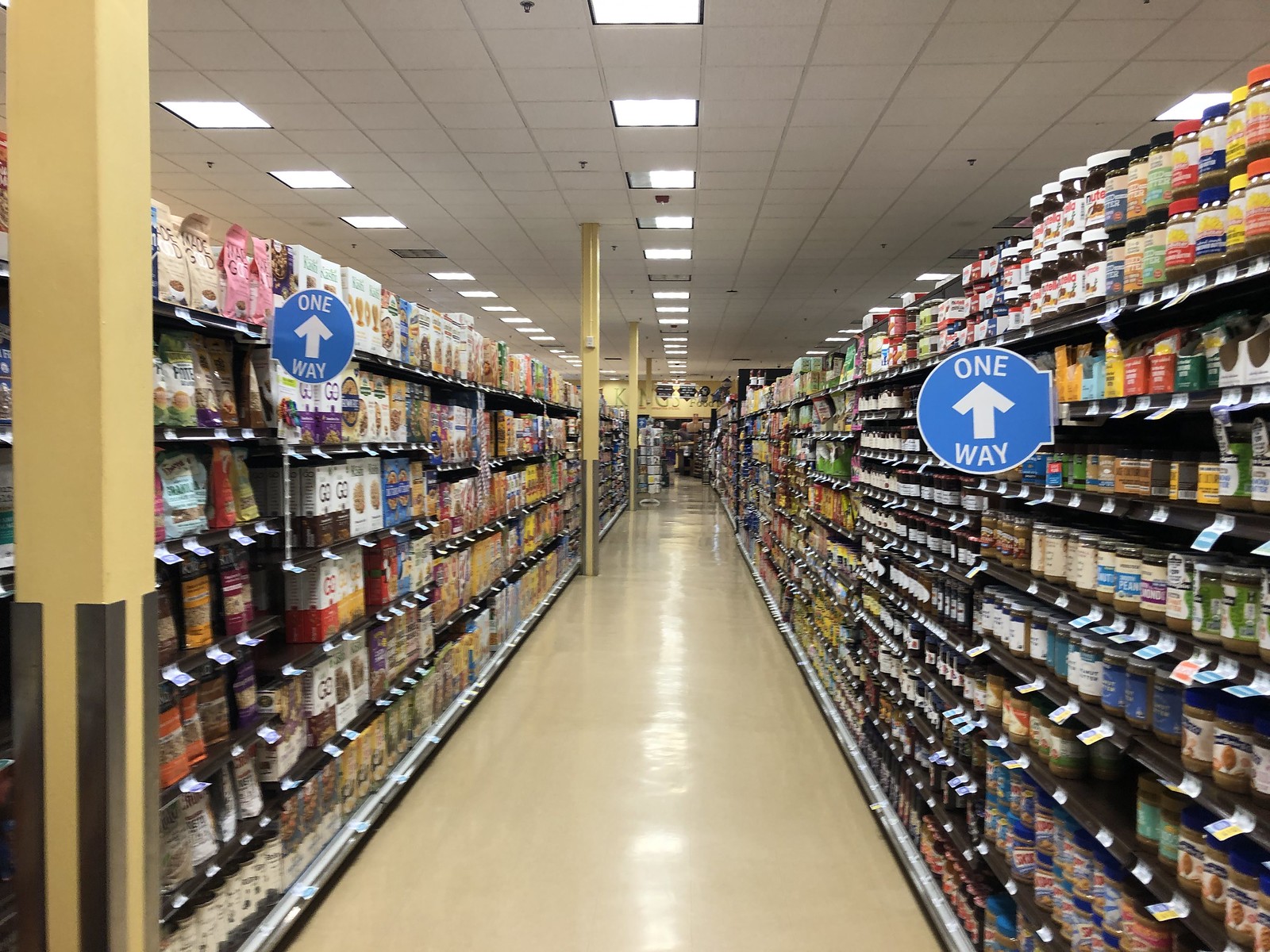The image depicts a meticulously organized supermarket aisle with a polished, reflective tile floor that is devoid of grooves, aiding in easy cleaning. Dominating the scene are blue signs on either side of the aisle, each labeled "One Way" in white letters with arrows pointing away from the camera to regulate the flow of shoppers, ensuring no backtracking or U-turns. The left side of the aisle features shelves filled with various dry goods, including brightly colored cereal boxes and snack packages in hues of white, blue, yellow, pink, and beige. Yellow posts rise from the ground to the ceiling on this side, their bases protected with black corner guards to prevent damage. On the right, shelves are stocked with an array of spreadable products such as Nutella and peanut butter, housed in jars with labeling and icons in diverse colors like white, yellow, red, purple, and green. The ceiling above is lined with multiple light tiles that evenly illuminate the aisle, casting bright reflections on the immaculate floor below.